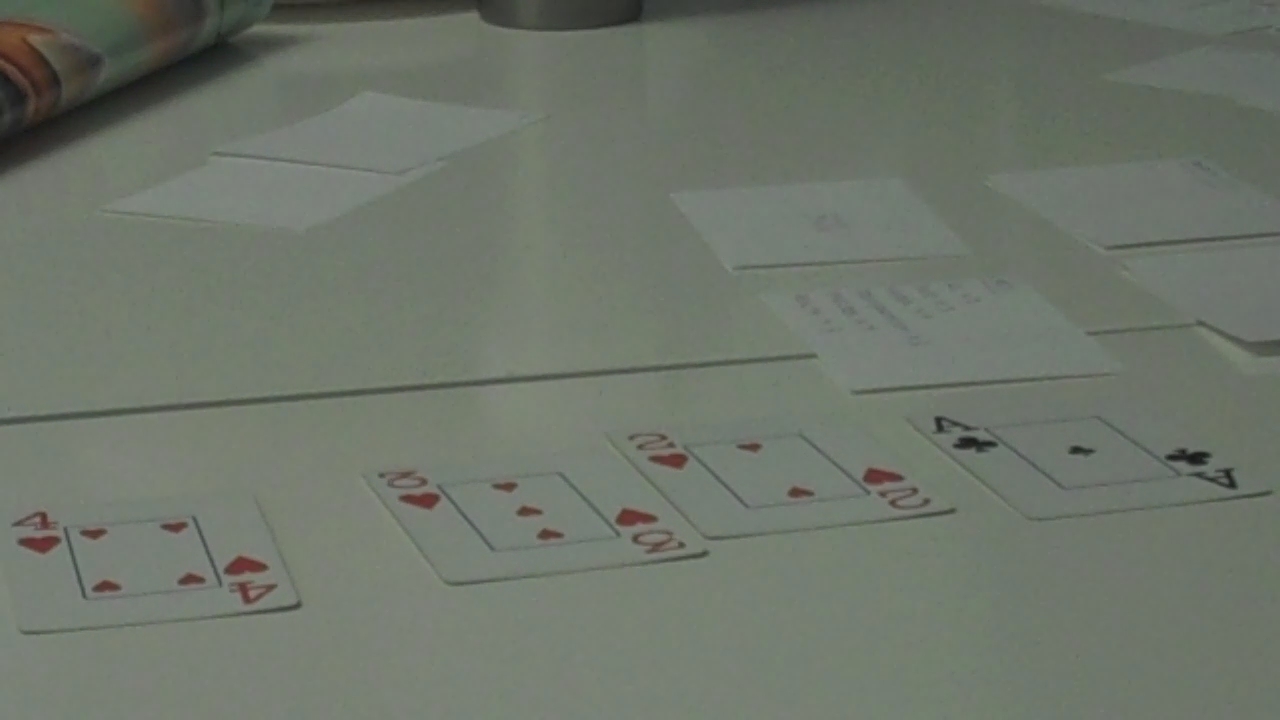On a white, foldable tabletop, a selection of playing cards and various small pieces of paper are spread out. The cards— the Ace of Clubs, the Two, Three, and Four of Hearts— are positioned nearest to the foreground. Scattered among them are several small notes: some blank, others partially or fully inscribed, including one that features a complete list. The table's surface shows a distinctive fold line running through the middle, indicative of its collapsible design. In one corner, a sliver of a rolled-up magazine peeks into the frame, while on the far side, the rounded base of a cup or similar object is visible. The playing cards appear to be moderately used, showing signs of handling but not extreme wear. The arrangement suggests a scene of casual gaming or a contemplative moment interrupted.